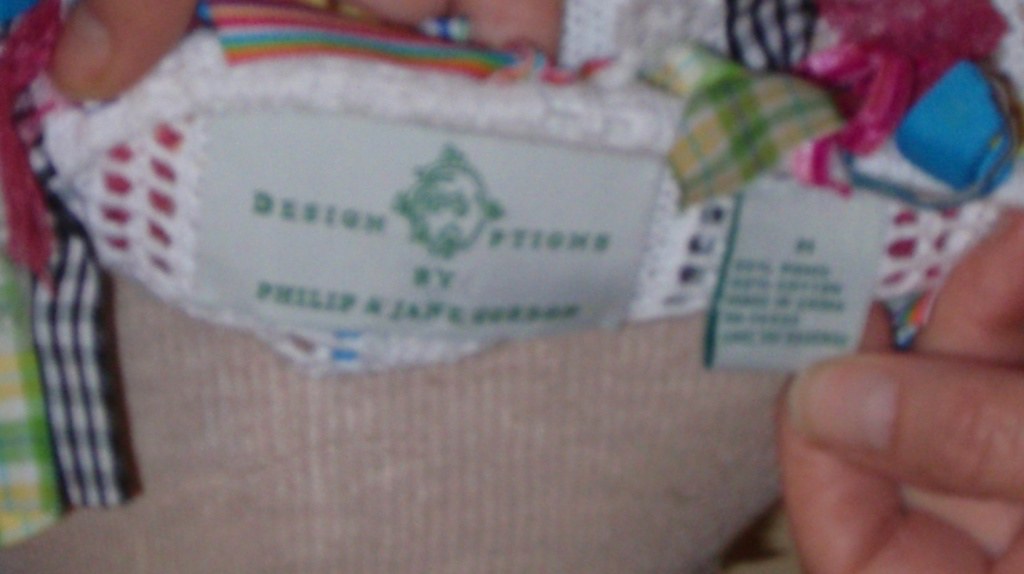This indoor, color close-up photograph captures a blurry and grainy image of two tags on a garment's collar, which appears to be a sweater or shirt with a white collar featuring red striping and a light tan lower half. Central to the image is a rectangular white tag with green lettering, partially legible, reading "design" and possibly "P-Town" or "Philip and somebody" below. Another hand-held tag is partially visible in the upper half of the image, specifically in the lower right corner, where someone's left thumb and index finger are attempting to display it. However, the text on this tag remains unreadable due to the image's poor focus. Surrounding the tags and clothing are various colorful ribbons, including blue and white plaid, green and yellow plaid, pink and white plaid, and a crocheted white strip, suggesting a mix of fabric patterns and textures. A slight glimpse of the person's other thumb appears in the upper left corner. The backdrop is either a sofa or bed covered with an assortment of fabrics.